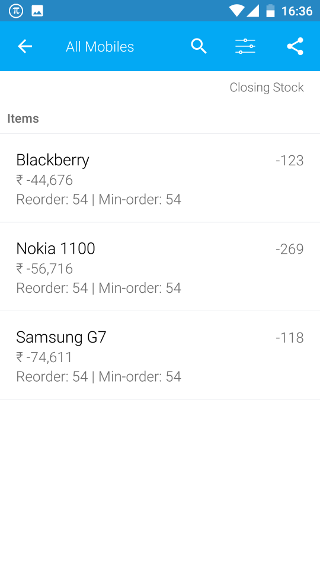The image is a detailed screenshot from a smartphone interface, captured at 16:36, as indicated by the white time display at the top-right corner of the screen. Adjacent to the time, the status bar exhibits a white battery icon showing approximately two-thirds charge, a triangle symbol representing wireless connection signal, and an inverted triangle for the Wi-Fi signal. On the top-left corner, there's a white square featuring a couple of tiny blue triangles, with adjacent icons, including a small circle and a stylized 'N' with a tilt.

Below this main blue border, there is a secondary turquoise border. On the left side of this border, a white arrow pointing left is displayed. Slightly left of the center, the words "All mobiles" are prominently written in white font. To the right, there's a search icon (a white circle with a line extending to the right) and a menu icon composed of three horizontal lines and three dots, followed by another icon with three connected dots.

The main background of the screenshot is white. On the left side of the screen, a list labeled "Items" is visible, presenting stock numbers for shares of different companies. The three companies displayed are BlackBerry, Nokia, and Samsung, each listed with their respective stock information.